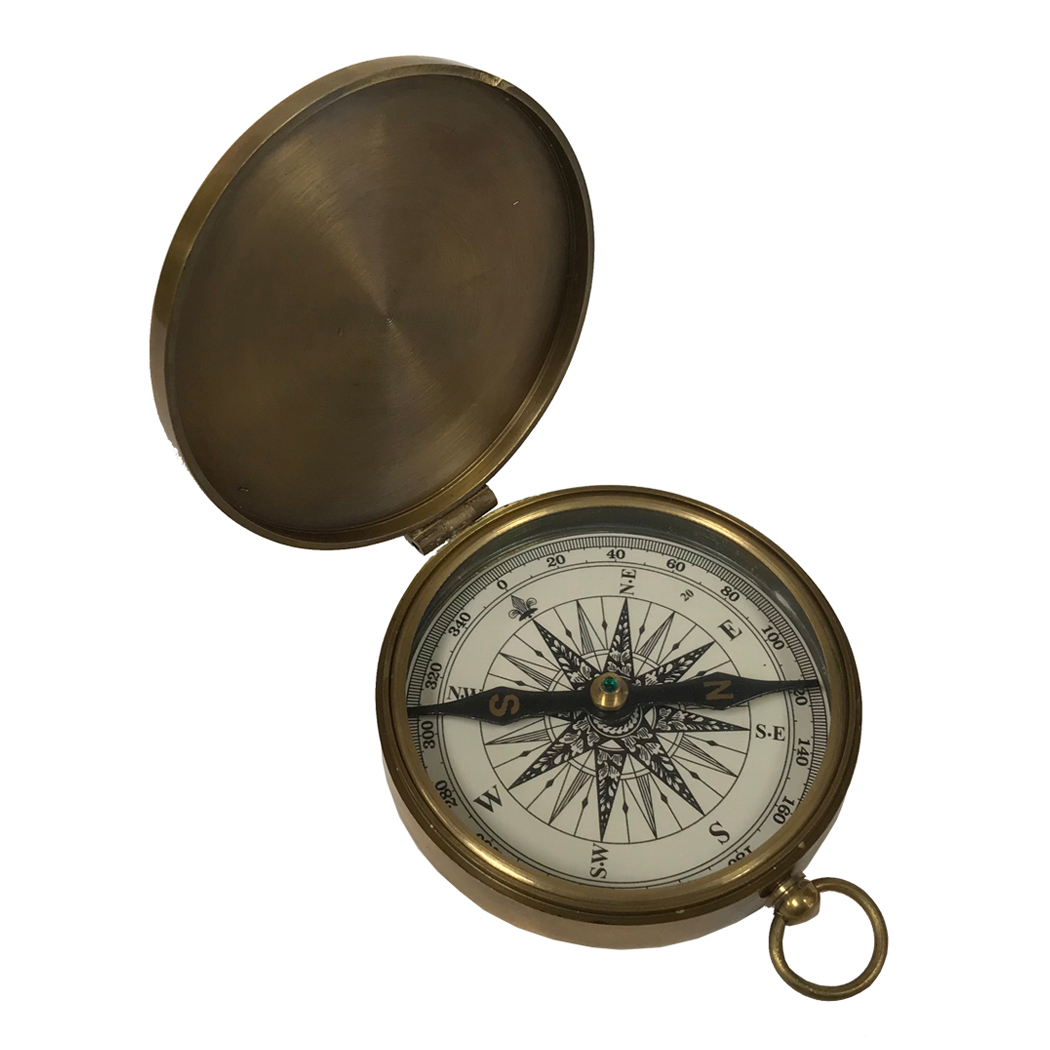The image depicts an antique pocket compass, resembling a pocket watch with a hinged lid. The compass is encased in a tarnished gold or bronze-like metal material, featuring an intricate design. The lid, which opens to reveal the compass, includes a small loop at the top for attaching to a keychain or chain, adding to its portability.

Inside, the compass face is predominantly white with crisp black text. Surrounding the face are degree markings starting at zero at the top center, and incrementing by 20, continuing around the circumference up to 340 degrees. The outer ring displays the cardinal directions, including North, Northeast, East, Southeast, South, Southwest, West, and Northwest. 

At the very center is a beautifully designed eight-pointed star. The compass needle, which is black, has the letters 'N' and 'S' in gold on its north and south points, respectively. This needle pivots around a central brass knob adorned with a small, green gem, adding a touch of elegance to the vintage aesthetic. The overall presentation, set against a clean, white background, highlights this compass as both a functional item and a piece of timeless design.